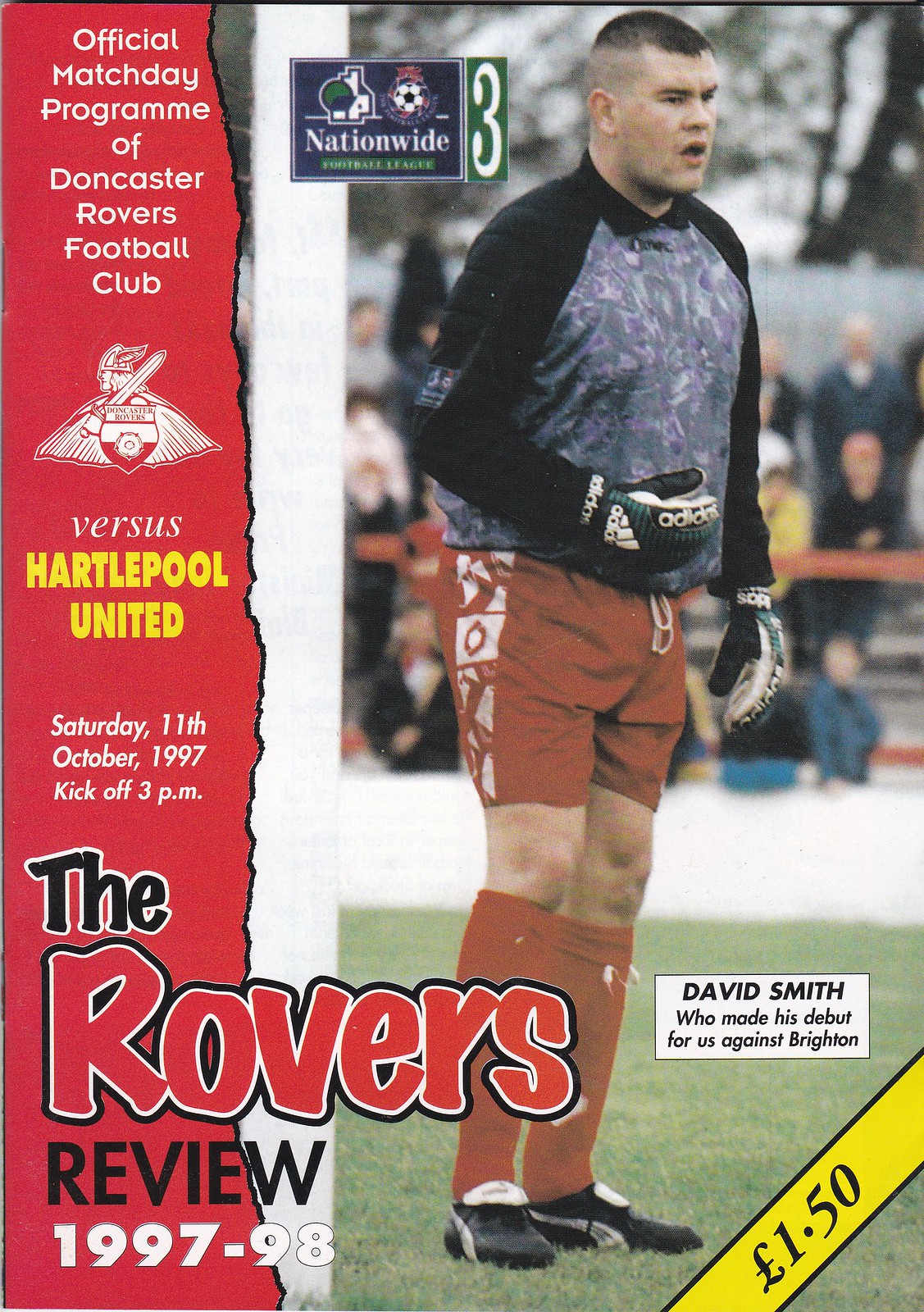This detailed cover photo of the Official Match Day Program for Doncaster Rovers Football Club features an image of goalkeeper David Smith, who made his debut against Brighton. He is depicted wearing a black long-sleeved shirt with blue and green mottling on the torso, red shorts, and red knee-high socks. David is standing on the grass and looking to the right. The left side of the cover prominently displays text in red, including the club's logo, indicating that it's Doncaster Rovers versus Hartlepool United on Saturday, 11th October 1997, with kickoff at 3 p.m. Below this, "The Rovers Review 1997-98" is printed in bold letters. A Nationwide Football League 3 logo is situated at the top center of the cover, while the bottom right corner features a white box with black letters highlighting David Smith's debut and a yellow price tag indicating a cost of £1.50. The backdrop includes spectators in the bleachers, suggestive of a cold day, potentially with snow on the trees.